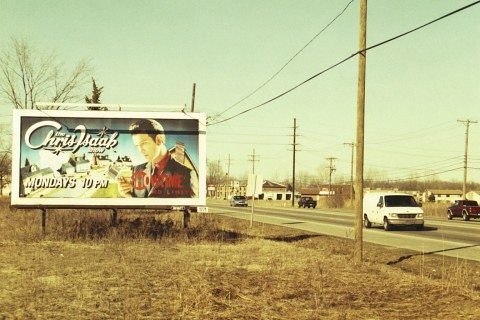The image features a large, cartoon-style billboard advertising "Chris Isaac," prominently displaying the text "Mondays at 10 p.m." The billboard is set against a backdrop of a deep blue sky with a brown house visible in the background. Chris Isaac is illustrated wearing a striking red and black outfit. The billboard is positioned low to the ground, surrounded by dead grass, and is flanked by a few trees. Above the billboard, there appears to be a light fixture, suggesting that it is illuminated at night. The scene is set along a relatively quiet road dotted with telephone poles. In the distance, a white building can be seen on the right side of the road, along with several houses. A few cars are visible, traveling in both directions on what appears to be a significant road for the area.